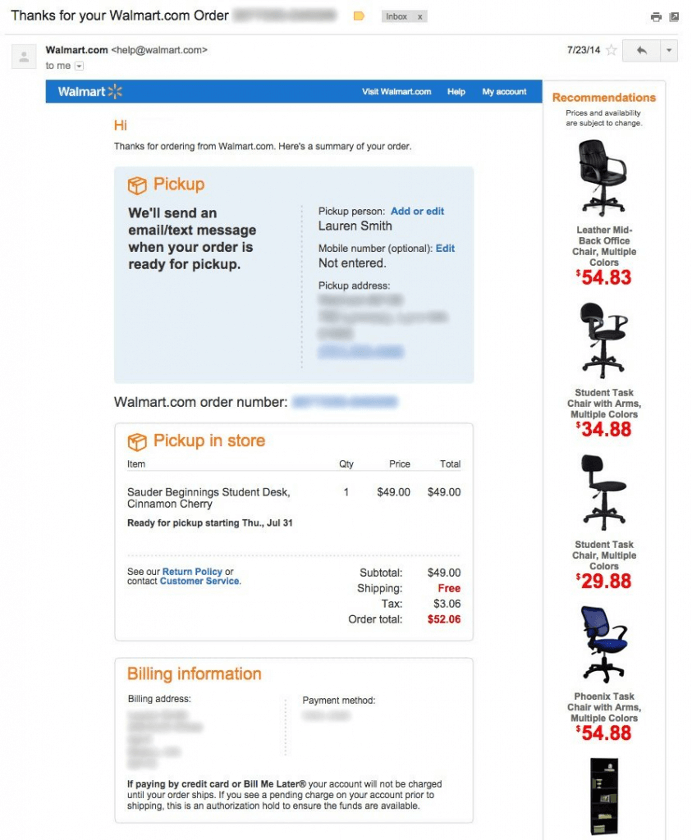**Caption:**

At the top of the image, in black text, it says "Thanks for your Walmart order." Below this text is a gray box with a green printer symbol beside it and a white arrow. A horizontal line separates this section from the text "Walmart.com," "help@walmart.com," and the date "7/23/14," all in black.

On the right side, there is a white star outline within a gray box and a gray arrow pointing to the left. Below this arrow, a triangle points downward. The background of this section is blue with a white border. In the white border, the text "Walmart" and the Walmart logo, which resembles an orange sun with radial lines, are prominently displayed. Additionally, "Visit walmart.com" is written in white text. Nearby, another white text reads "Help" followed by "My Account" in a smaller font. 

Further down, the word "Hi" appears in an arm-like font. Below that, the text says "Thanks for ordering from Walmart.com. Here's a summary of your order" in black. This is followed by a blue rectangle with an orange section on the left side labeled "Pick Up." In black, it states, "We'll send an email/text message when your order is ready for pick up." On the right side, under "Pick Up Person," the blue text "Add or Edit" appears next to the black text "Laura Smith, mobile number optional." Below this, "Edit" is in blue, followed by "Not Entered" in black.

Further down, the text in black reads, "Add a Pick Up Person." Next, the text "Walmart.com Order Number" is indicated but blurred out. The image proceeds with "Pick Up In-Store" followed by headings "Item," "Quantity," "Price," and "Total."

The first item listed is "Student Desk Cinnamon Cherry," ready for pick up starting Thursday, July 31st, at a price of $49, making the total $49.